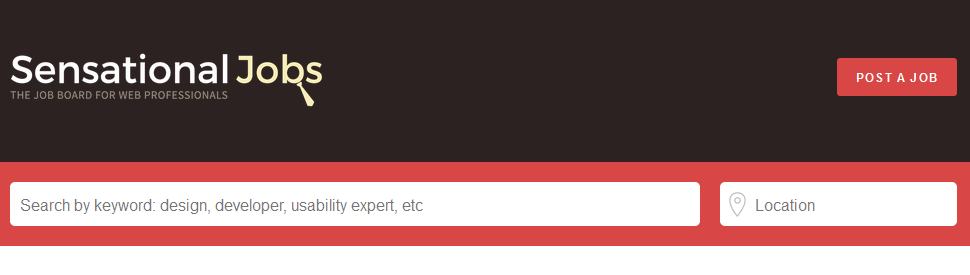The image depicts a rectangular job search website with a primarily black background, significantly wider than its height. Spanning across the top left section of the page, the word "Sensational" appears in white text, followed by "Jobs" in a beige color, both set against the stark black background. Directly beneath this, in all capital letters and a medium gray font, the phrase "THE JOB BOARD FOR WEB PROFESSIONALS" is displayed, though the contrast makes it somewhat difficult to read.

Below this tagline, a prominent red rectangle extends horizontally across the width of the page. Within this red rectangle is a white rectangular box containing a searchable field with the placeholder text, "Search by Keyword: Design, Developer, Usability Expert, etc." Adjacent to this search box, on the right-hand side, lies another white box labeled "Location."

In the upper right corner of the page, a striking red rectangle catches the eye. Inside this rectangle, in white, all-capital letters, is the call-to-action button labeled "POST A JOB."

Aside from these elements, the page remains uncluttered and devoid of additional text.